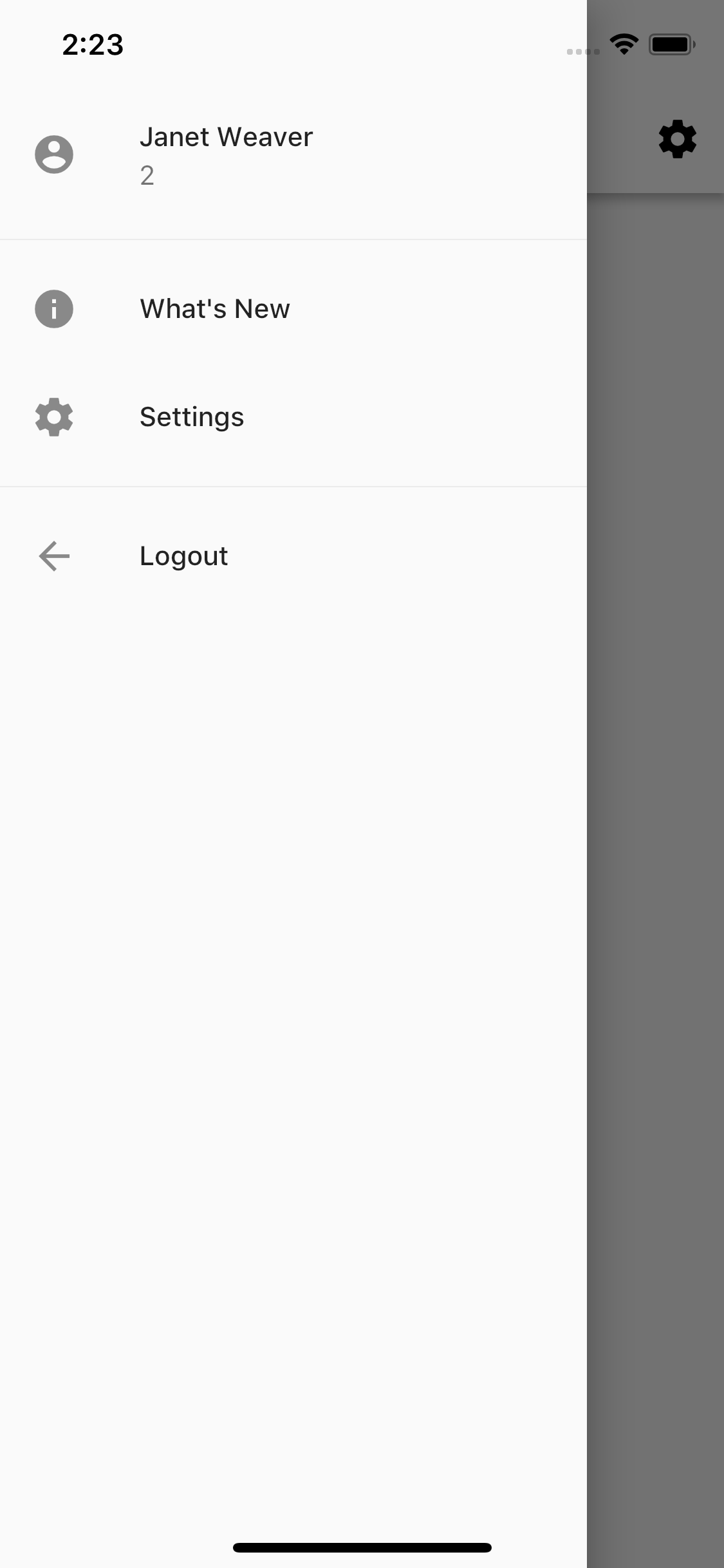The image depicts a phone menu screen that is divided into two distinct sections. The left two-thirds of the screen display a prominent overlay menu, while the right third of the screen appears faded and dark, revealing the underlying interface.

In the top-left corner of the overlay menu, the time "2:23" is clearly visible. Directly below the time, there is a profile icon represented by a circle containing a human silhouette, with the text "Janet Weaver" adjacent to it. Beneath the profile icon, an eye icon in a black circle is present, accompanied by the label "What's New." Below this, a gear icon is seen with the label "Settings" next to it. Further down, there is a left-pointing arrow icon, with the text "Log Out" to its right.

On the faded right side of the screen, there are three icons located in the top right corner: a Wi-Fi icon, a horizontal battery icon, and a settings gear icon.

Finally, at the bottom of the image, a black horizontal scroll bar is centrally placed, spanning across the lower portion of the screen.